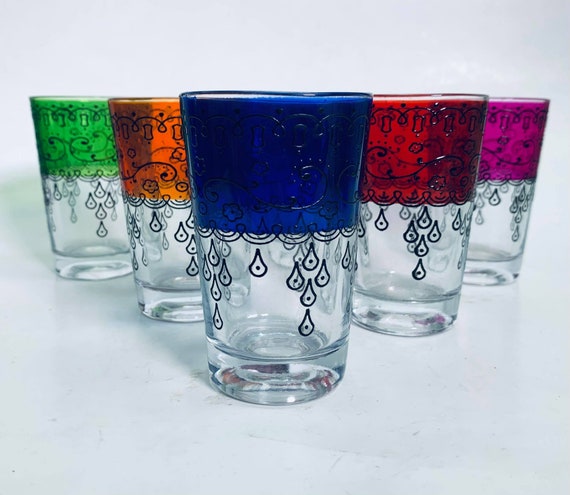The photograph captures five tall shot glasses arranged in a pyramid-like pattern on a light gray background. Each glass features intricate Hanna-style designs with black teardrop-like shapes dripping down the clear bottom half. The top halves are vividly colored and each glass sports a different hue: blue, orange, red, pink, and green. The layout shows one blue glass at the forefront, flanked by an orange glass to its left and a red glass to its right, while a green glass and a pink glass form the back row. The background seamlessly blends with the smooth surface, creating a striking contrast that highlights the colorful upper halves of the glasses.